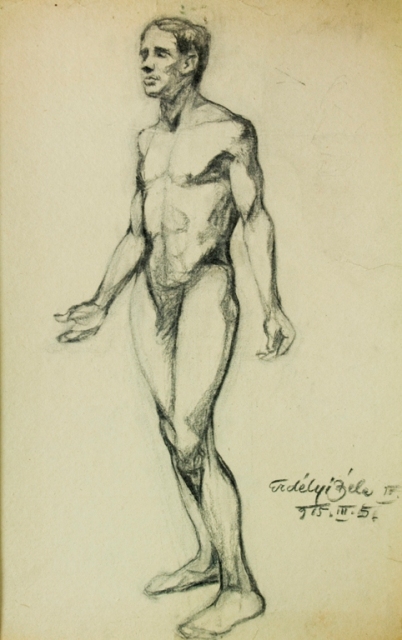This image is a highly realistic pencil or charcoal drawing of a nude man, centrally positioned against a solid white background. The paper itself is aged, showing yellow-brown stains at the corners. The man, depicted with meticulous attention to detail, stands upright, with both arms down and palms open to the sky. His feet are placed side by side. The drawing captures the toned musculature of his stomach and chest, making it lifelike and evocative of a study in anatomy. The artwork primarily uses shades of black, white, and gray, with an overall sepia tone due to the paper's aging. In the bottom right corner, there's an illegible signature in black, possibly accompanied by a date. The sketch-like areas, particularly his right hand on the left-hand side of the image, contrast with more defined sections, indicative of a work-in-progress or a practice piece from an art class.